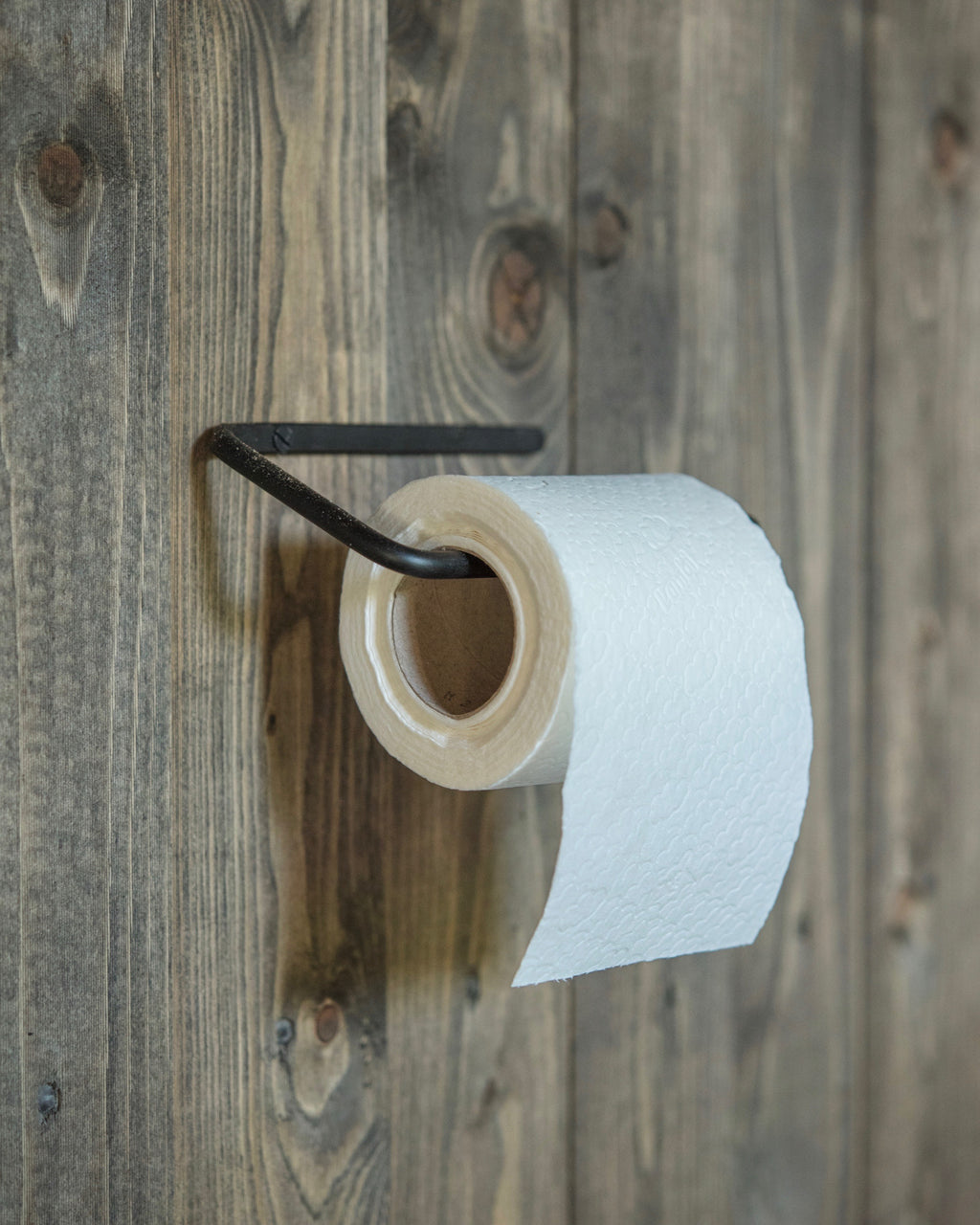The image portrays a simple yet detailed scene centered around a toilet paper holder mounted on a wood plank wall. The wall itself is made of finely finished, beige and dark wood grain panels, displaying varying shades of brown, from dark to light. The wall also features rusted reddish screws, hinting at their original black color, securing the planks in place.

The toilet paper holder is crafted from black wrought iron, bent into a sharp and minimalistic C or U-shape, and is fixed to the wall with two black screws. The roll of toilet paper hanging from the holder appears flimsy and almost empty, with the paper unfurling over the top and hanging to the right. The stark contrast between the dark, rustic wooden wall and the black iron holder emphasizes the understated simplicity of the scene, while the nearly depleted roll of toilet paper adds a touch of everyday realism.